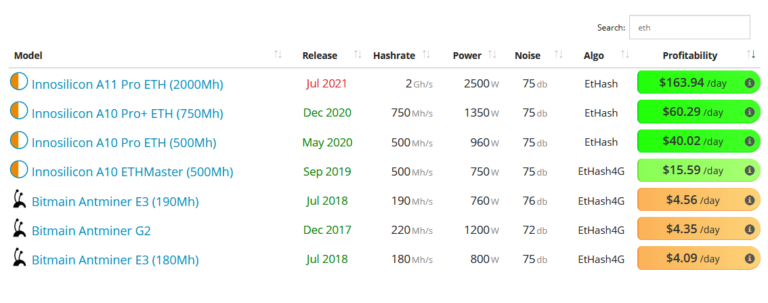The image is a detailed screenshot of a cryptocurrency mining comparison table. In the top-left corner of the screen, the word "Model" is prominently displayed in bold black text. To the right, the categories "Release," "Hashrate," "Power," "Noise," "Algo," and "Profitability" are listed. Above these categories is a search bar with the word "Search" beside a white rectangular input field edged with a gray border, containing the text "ETH" aligned to the left.

Under the "Model" category, there are several entries, each represented by a semi-circular icon split into orange and gray segments. The first entry is labeled "Innosilicon A11 Pro ETH (2000MH)," with corresponding data under the other categories such as release date, hashrate, power consumption, noise level, and algorithm profitability. Subsequent entries follow the same format, including "Innosilicon A10 Pro+ ETH," "Innosilicon A10 Pro ETH (500MH)," and "ETH Master (500MH)." Each model presents its unique data under the associated categories, accompanied by distinct icons to their left. Additionally, Bitmain Antminer models are listed three times, each adhering to the same structured format.